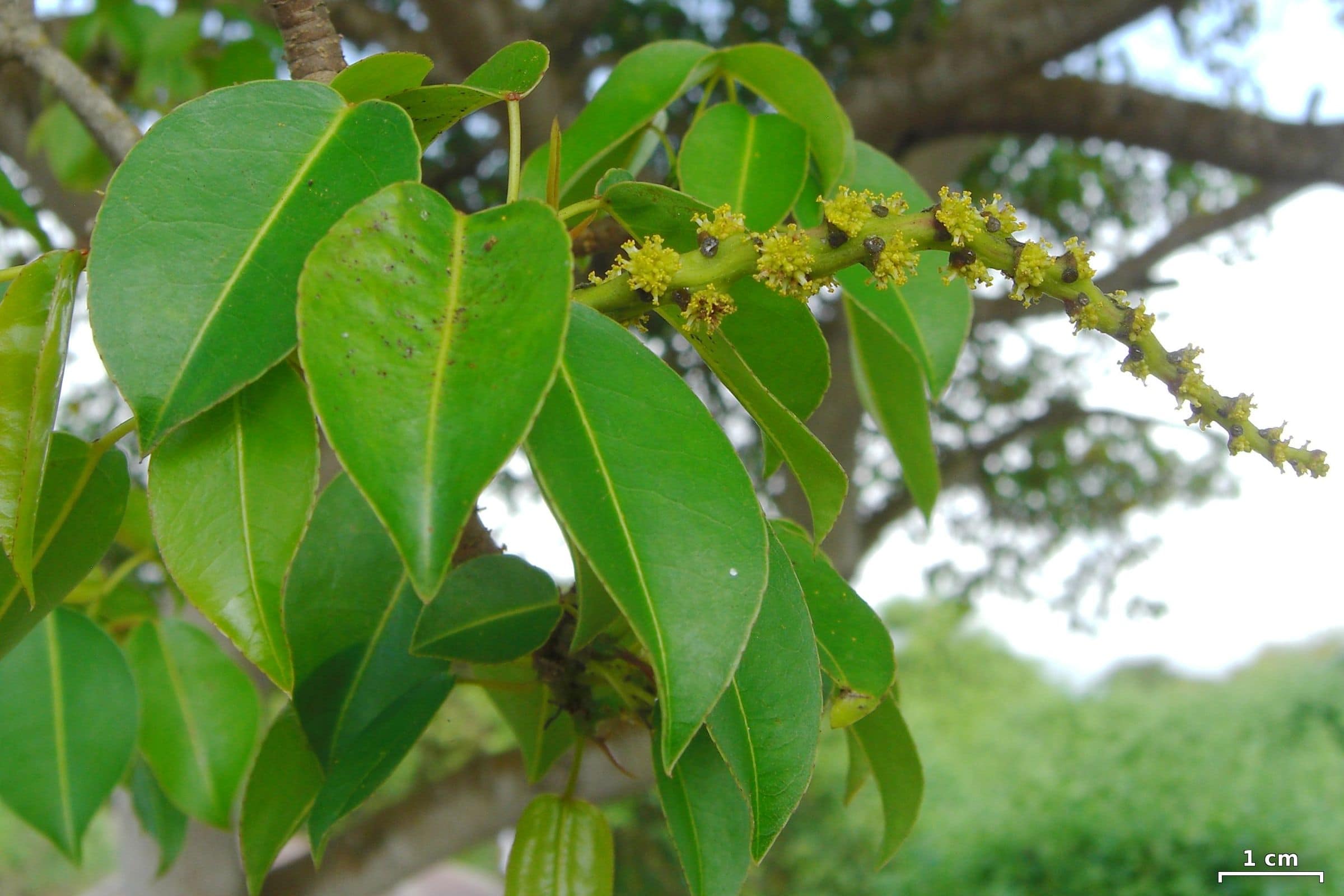The image depicts a close-up view of a tree with heart-shaped leaves. The leaves hang from a dark gray-brown branch and are seen against a backdrop of a bright blue and white sky, indicating daylight. The main focus is on the leaves, which have a light green vein running down the center, giving them a slightly drooping appearance. In the center of the cluster of leaves, a slender, light green twig extends outward and then gently curves back. This twig is adorned with tiny black dots, from which clusters of very small, light green leaves and yellow pointy buds emerge. The background features more dense, green foliage, adding depth to the image. Additionally, a watermark with a scale indicator, marked "1 centimeter," is visible in the bottom right corner, emphasizing the detailed nature of the photograph.